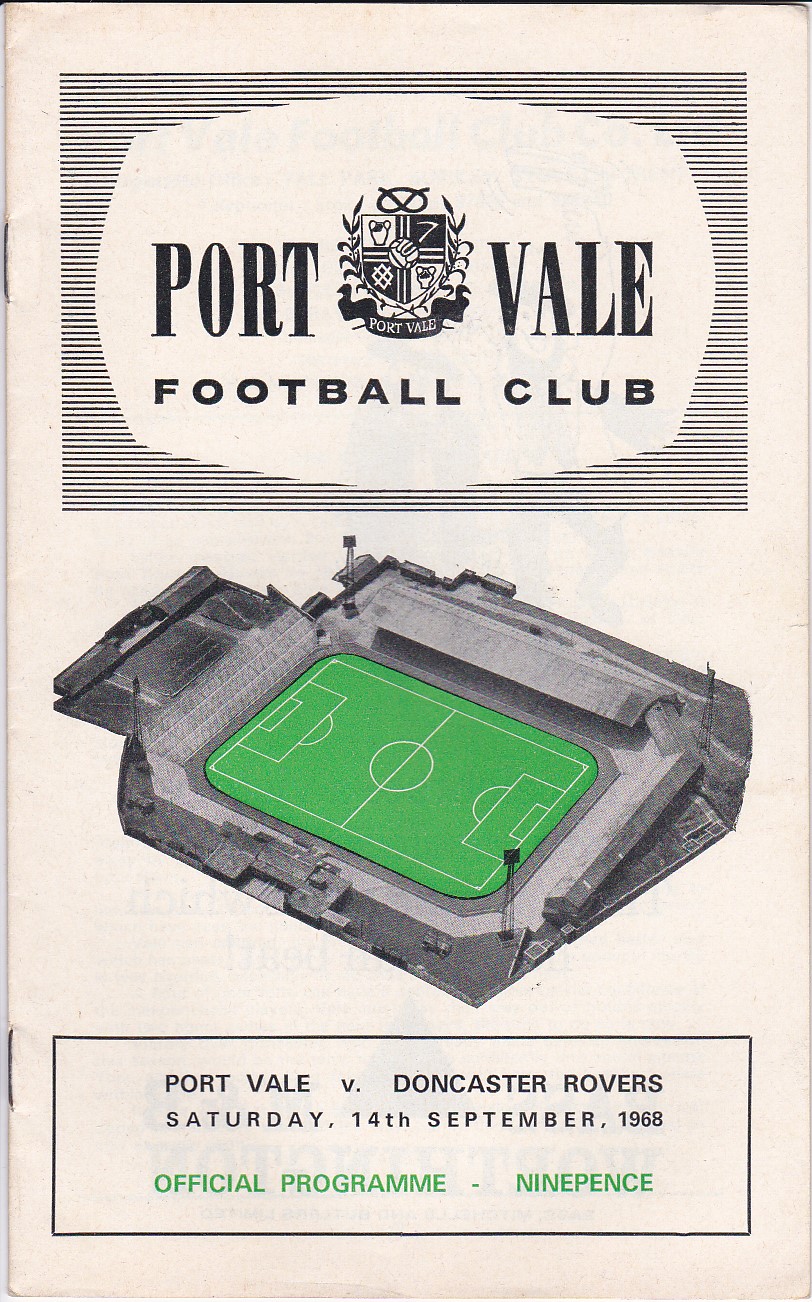The image showcases a scanned, aged program from Port Vale Football Club, dating back to September 14, 1968. The background has a tan hue due to the old paper. At the top, "Port Vale Football Club" is prominently displayed, accompanied by a black-and-white insignia featuring a shield with a soccer ball and a pretzel-like logo, giving it an off-white appearance. Centered in the image is a green soccer field, surrounded by black and white tones. Below the field, the text reads, "Port Vale vs. Doncaster Rovers, Saturday, 14th September 1968, Official Programme," with a cost of nine pence. The program is staple-bound, resembling a pamphlet typically handed out at the entrance of a soccer game, preserving the match's historical essence.